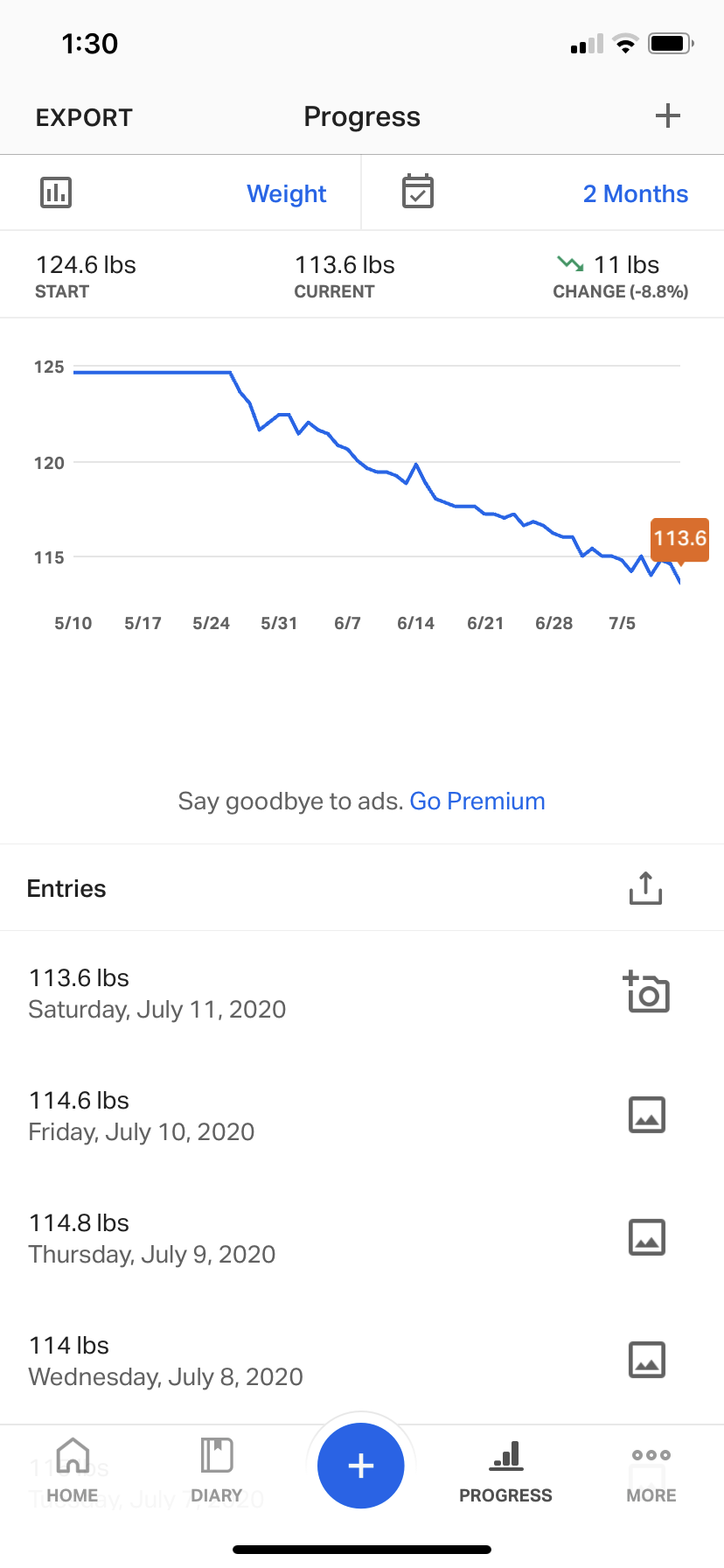This detailed screenshot from a person's cell phone displays their weight loss progress over a span of two months. At the top of the screen, a timestamp reads "1:30" on the left, while the right side shows icons for coverage, Wi-Fi, and battery status. Below this, there are menu options labeled "Export," "Progress," and a plus sign. 

The main interface includes a weight tracker starting at "124.6 pounds" and currently at "113.6 pounds," indicating a loss of "11 pounds" which is noted as a "minus 8.8% change." A graph dominates the screen, featuring a spiky blue line that initially remains flat before descending to the bottom. Vertical markers along the left edge read "125," "120," and "115." Horizontal date markers include "5/10," "5/17," "5/24," "5/31," "6/7," "6/14," "6/21," "6/28," and "7/5." At the graph's endpoint, an orange square highlights the figure "113.6."

Beneath the graph, a prompt encourages users to "Say goodbye to ads, go premium." The entry log follows, listing weight recordings as:
- "113.6 pounds, Saturday, July 11th, 2020" with a camera icon,
- "114.6 pounds, Friday, July 10th, 2020" with a picture icon,
- "114.8 pounds, Thursday, July 9th, 2020" with a picture icon,
- "114 pounds, Wednesday, July 8th, 2020" with a picture icon.

The bottom navigation menu includes options labeled "Home," "Diary," "Progress," and "More."